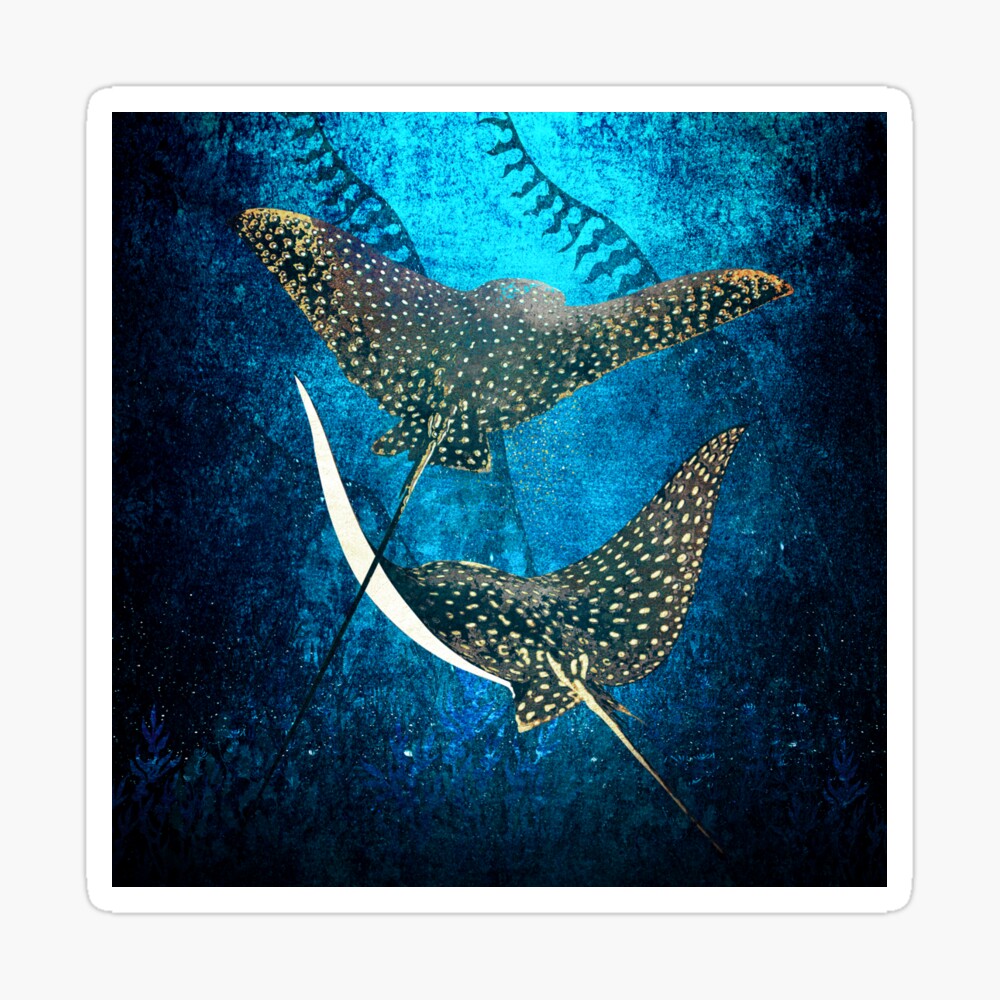This large square image, resembling a detailed piece of artwork, depicts an aquatic scene set against a light gray background framed by a white border. The central part of the image features a textured gradient of blue, transitioning from a light blue in the middle to a darker blue, almost black, on the sides, interspersed with tiny white speckles evoking the look of a starry sky. Two dark gray lines, reminiscent of stitching on a baseball, descend from the top across the light blue area.

In the center, two large creatures that appear to be stingrays - though at first glance they might be mistaken for birds or angel fish - dominate the scene. These stingrays are black or dark brown, adorned with gold or yellow polka dots suggesting a resemblance to whale sharks. Their distinctive, long, pointed tails start brown and fade to black. The stingrays are positioned one above the other, facing in opposite directions, with the lower one's tail extending towards the lower right and its white undersides visible. The light blue water surrounding them seems almost designed, raising questions about whether this effect is a natural underwater scene, an artistic addition, or perhaps indicative of an aquarium setting. Overall, the image merges elements of realism and art to create a captivating underwater tableau.